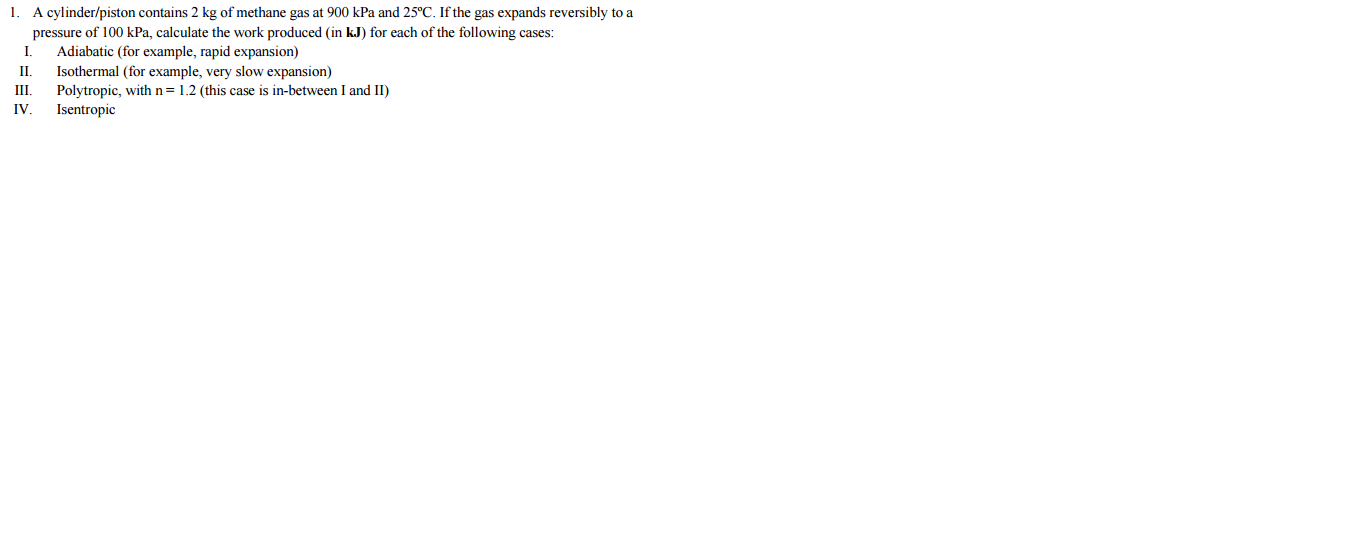Sure, here is a cleaned-up and detailed caption for the given image:

---

A physics problem is presented against a mostly white background. The problem states: "A cylinder/piston contains two kilograms of methane gas at 900 kPa and 25 degrees Celsius. If the gas expands reversibly to a pressure of 100 kPa, calculate the work produced in kilojoules for each of the following cases:

1. Adiabatic (e.g., rapid expansion).
2. Isothermal (e.g., very slow expansion).
3. Polytropic with n = 1.2 (this case falls in between adiabatic and isothermal).
4. Isentropic."

The text outlines the initial conditions and the various methods for calculating the work produced during the expansion of the gas.